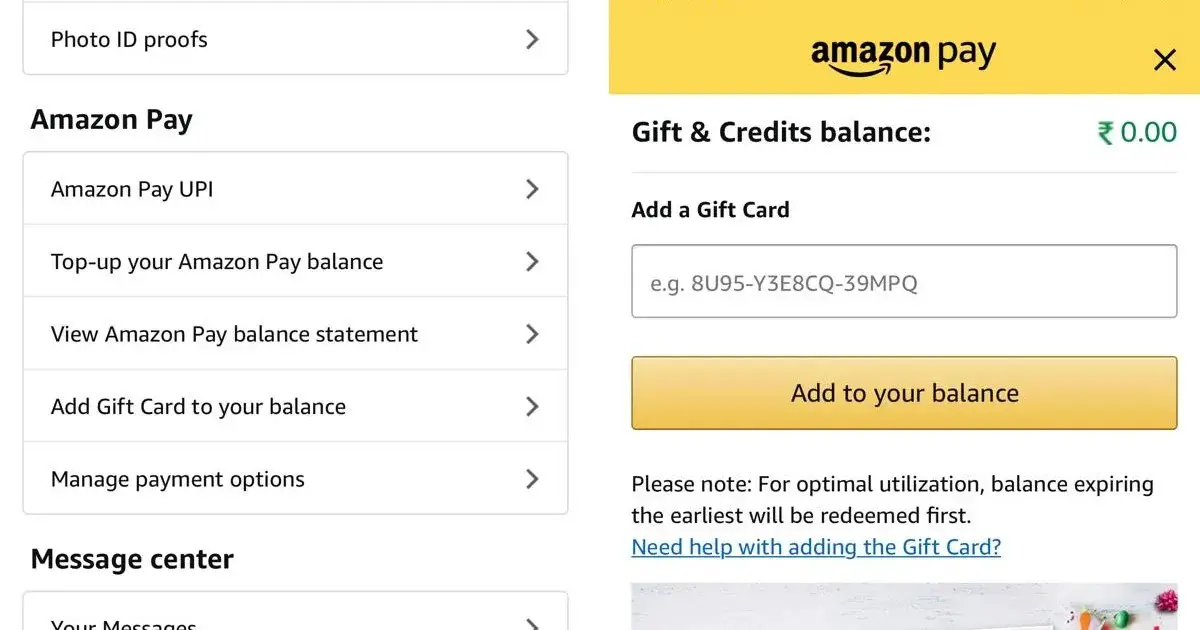The image is a left-to-right horizontal screenshot with a white background, presumably from a computer screen. On the upper left corner, there is a slim, grey rectangular box outlined in black with the label "Photo ID Proofs" and a clickable arrow next to it. Directly beneath, in bold black text, it states "Amazon Pay."

Below this section, a larger rectangular box is divided into five slots separated by grey horizontal lines, each containing various Amazon Pay options. The options are listed in black text, starting with "Amazon Pay UPI," followed by:
1. "Top up your Amazon Pay balance"
2. "View Amazon Pay balance statement"
3. "Add gift card to your balance"
4. "Manage payment options"

The fifth slot is labeled "Message Center," in bold black, though the phrase "Your Messages" appears cut off.

On the right side of the image, there is a long yellow rectangular box featuring "Amazon Pay" in black text with a small "X" in the corner. Below this, the section labeled "Gifts and Credit Balance" shows an amount in a different currency denomination reading "0.00." Below this amount, there is an input box to add a gift card number, accompanied by a darker yellow box labeled "Add to Your Balance." There is also an option to click for help with adding a gift card.